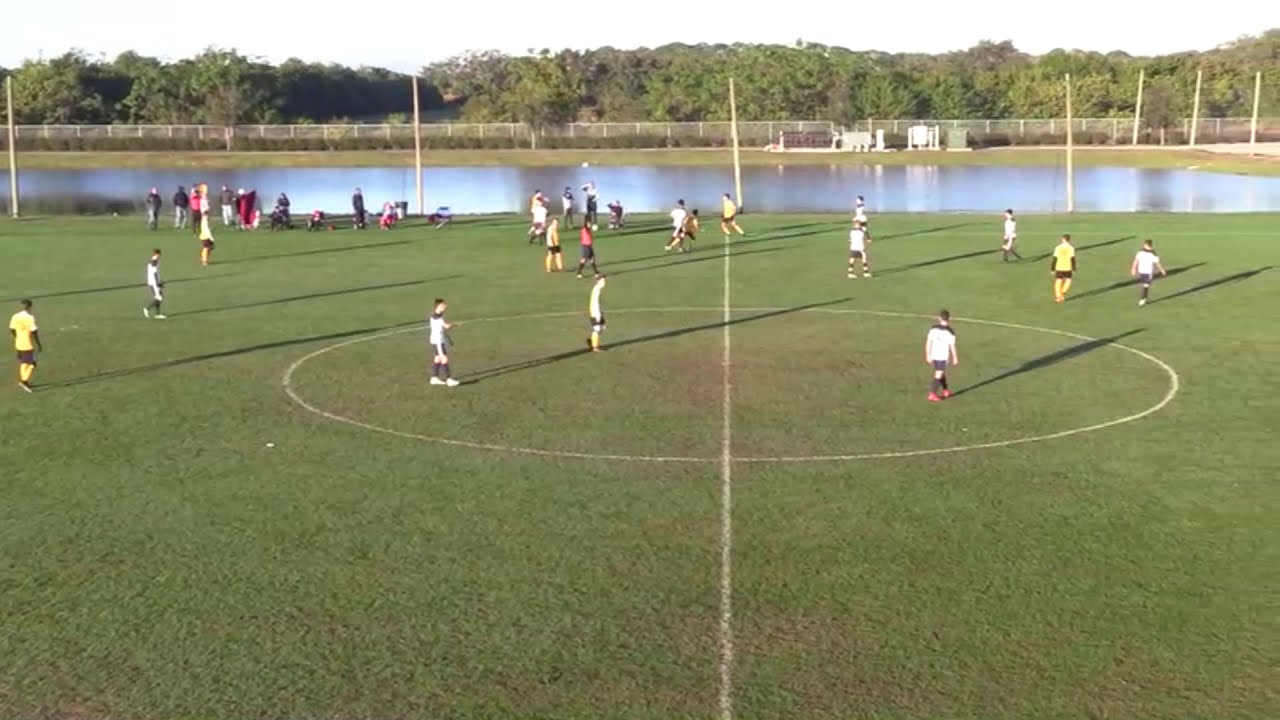In this elevated, overhead view of a youth soccer match, the scene captures a grassy soccer field marked by a prominent white half-court line and center circle. Two teams, distinguishable by their yellow and white jerseys paired with dark shorts, engage in the game predominantly on the far side near the midfield. Long, left-to-right shadows suggest late afternoon sunlight, casting elongated player silhouettes across the field. In the background, a large, blue pond reflects the bright, washed-out sky, bordered by a white fence, hedge shrubs, and a line of trees. On the far sidelines, scattered spectators and perhaps a few power poles are visible. The action seems to be gearing up for a possible throw-in, with players poised for movement.